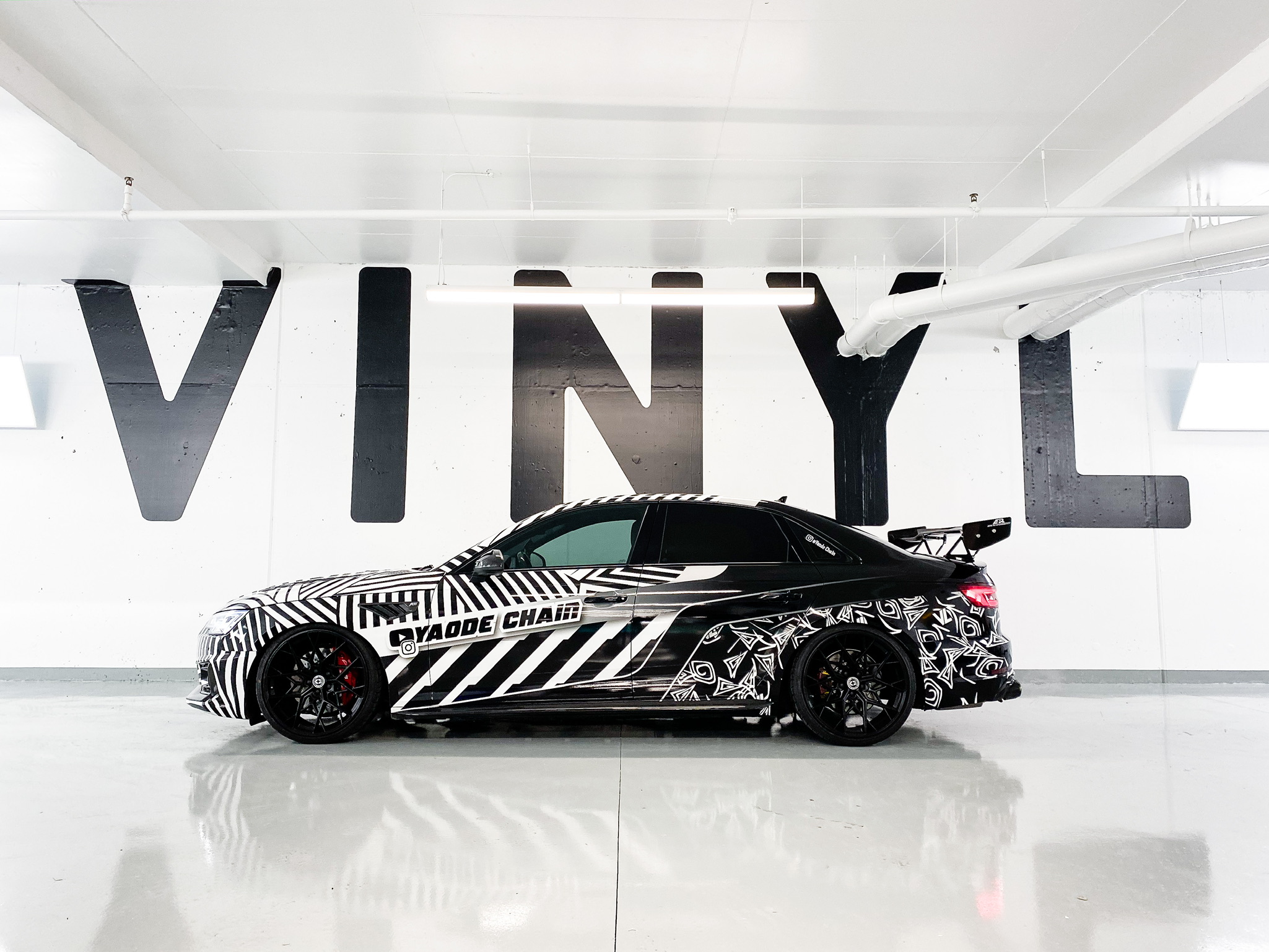This photograph showcases an intricately decorated sports car in a brilliantly illuminated showroom. The room features an extremely shiny, reflective white tiled floor that enhances the overall brightness. Along the back wall, large black rounded text spells out "VINYL," set against a pristine white backdrop. The right side of the frame includes two sets of white pipes and a white tube running horizontally from the ceiling, supporting a single bar of white light. The car, adorned with an elaborate black and white vinyl wrap, is positioned sideways facing left. The design includes black and white stripes across the hood, intersected by a black YouTube logo and text reading "YADA chain." The side features flowing black and white patterns with embedded white triangles, while the car’s rear sports a black spoiler. Black tires with matching rims and window frames complete its striking, zebra-striped appearance.